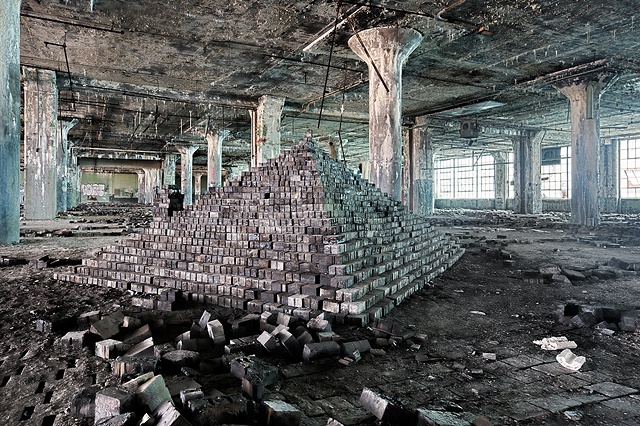The photograph captures the interior of a derelict, industrial building, possibly an old parking garage or warehouse, now in a state of extreme disrepair. The expansive space is dominated by floor-to-ceiling cement pillars that support a cracked and partially destroyed ceiling. Piles of scattered bricks cover the floor, with a conspicuous pyramid stack of these bricks standing as the focal point. Graffiti adorns one of the walls on the left side of the image, adding to the sense of neglect. Hanging electrical wires, a damaged air conditioning unit, and various metal pieces dangle from the ceiling, contributing to the chaotic and ruined atmosphere. The overall scene is one of utter destruction and mess, with elements suggesting the aftermath of a fire or extensive demolition work.